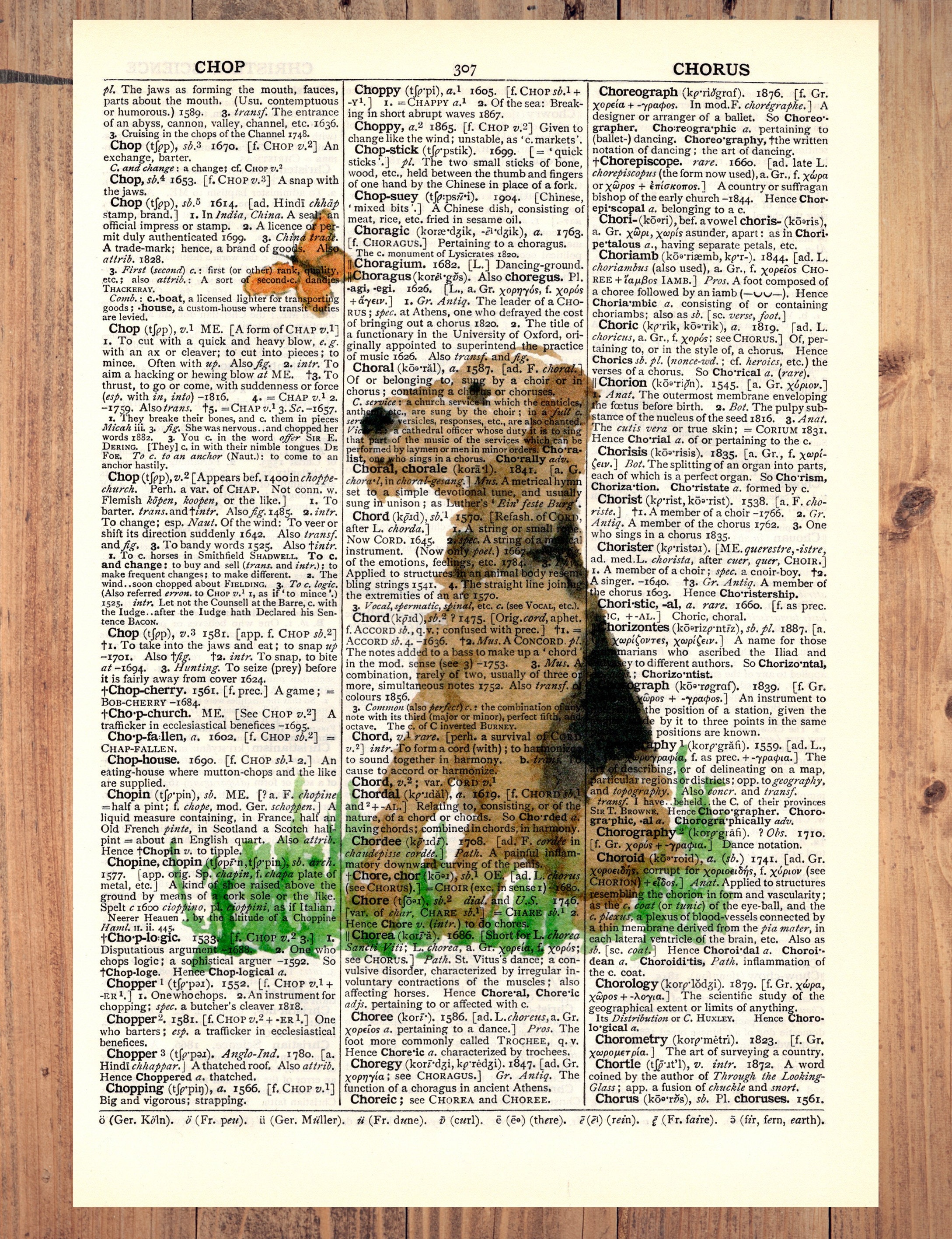The image depicts a page from a printed encyclopedia, identified as page 307, laid atop a background of wooden planks. The page features three vertical columns of densely packed black text, resembling dictionary entries, with the word "CHOP" and various derivations prominently listed at the top. Inscribed at the top of the third column is the word "CHORUS." Overlaying this text, the page serves as a unique canvas for an acrylic painting of a terrier dog. The dog, resembling an Airedale or a large terrier, is painted in tones of brown with distinctive black markings on its neck and back. The dog is seated in a patch of green grass, intently gazing at an orange butterfly trimmed in black, hovering just out of reach above its nose. This charming and whimsical scene juxtaposes the structured information of the encyclopedia with lively and colorful artwork.